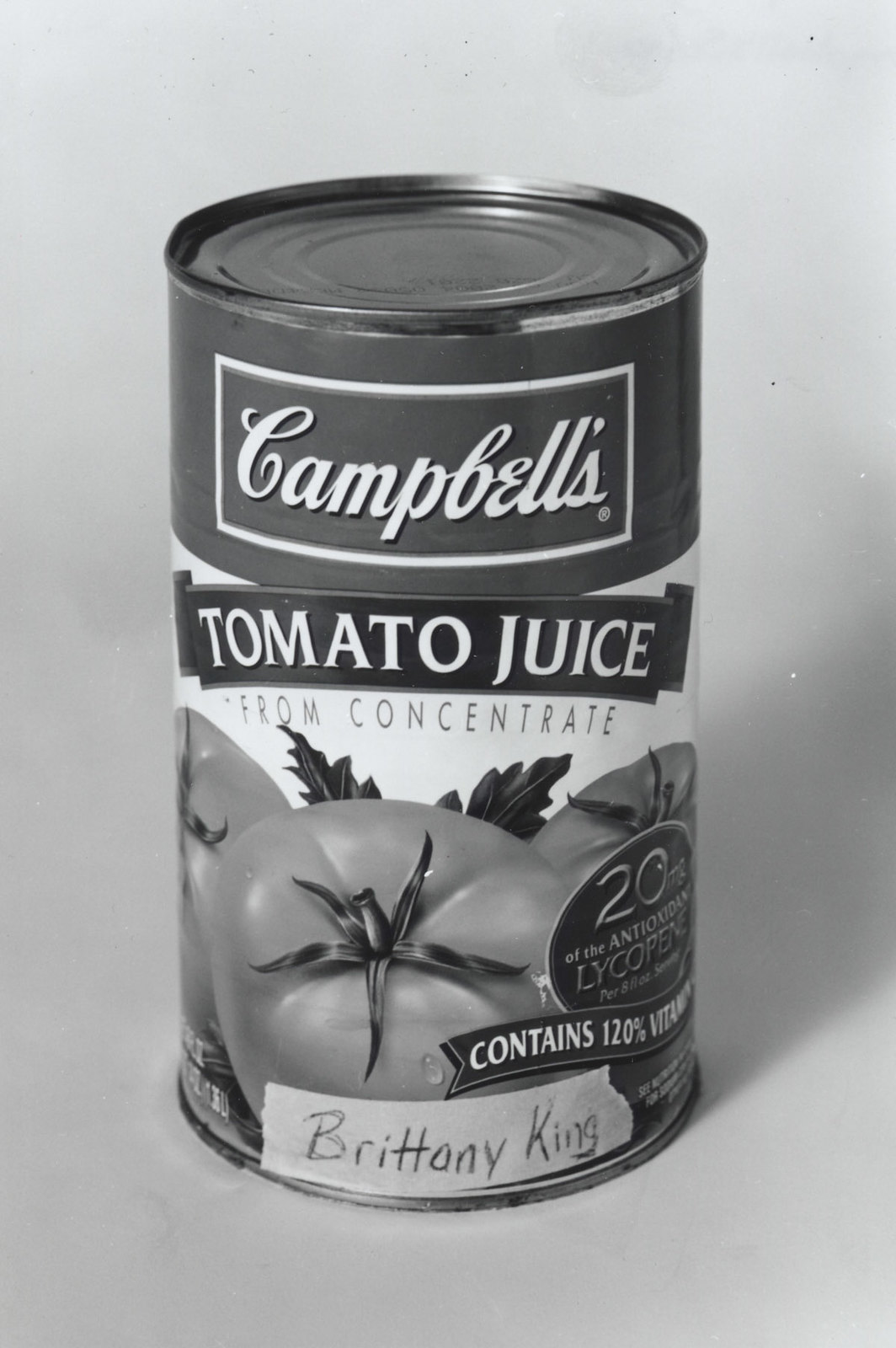This black and white photograph showcases a Campbell's tomato juice from concentrate can as the central object. The can features a distinctive design with a solid label at the top, and the iconic "Campbell's" script in a white rectangular outline. Below that, the dark banner prominently displays the words "Tomato Juice" in white text, with "From Concentrate" written beneath on a white background. The can is adorned with realistic images of ripe tomatoes, complete with leaves, and a notably detailed depiction of a large tomato in the center, which has two leaves and a stem with five petals. The can's label includes several pieces of information, such as "120% vitamin" though the exact details are partially obscured. Additionally, there's a piece of brown tape at the bottom with the name "Brittany King" written on it. The background is a neutral white that appears grey due to the black and white nature of the image, enhancing the classic and nostalgic feel reminiscent of traditional Campbell's soup can designs.